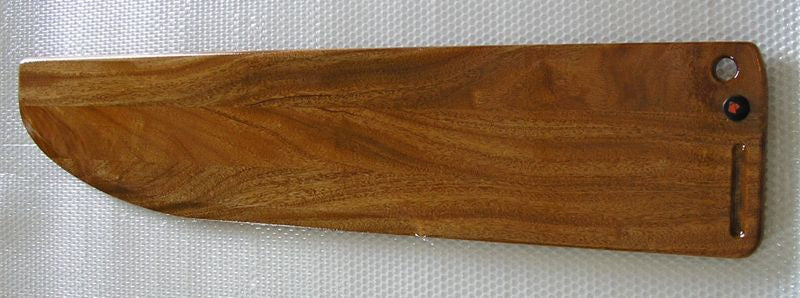The image depicts an almost blade-shaped wooden object mounted on a flat, white surface. The piece, made of multiple types of wood with intersecting grains, measures approximately six inches in length and two and a half inches in width. The left side features a curved, cut-out section resembling a knife’s edge, while the right side shows notable details: a slit and two holes—a drilled hole near the top and a black button or circular mark below it. The object has a sharp, slightly undulating edge from left to right, giving it a boat-like appearance. Though it looks like a thin cutting board or paddle, its exact purpose remains unclear.